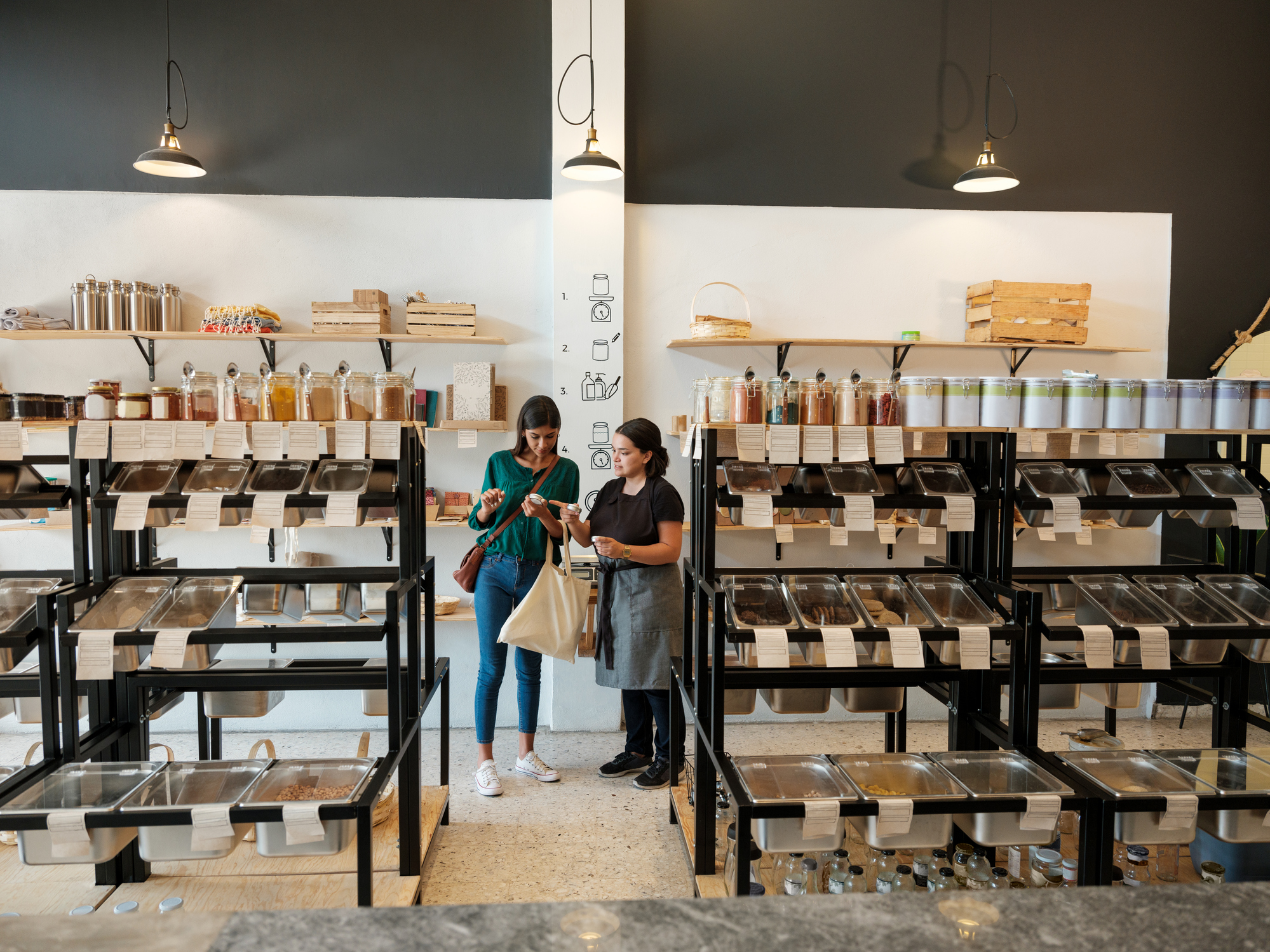In the image, two women are inside a brightly lit health food store, distinguished by its white and gray walls and white tiled floor. The store is well-organized with various round, shallow containers on shelves, each filled with different colored dry goods and spices, neatly labeled but unreadable in the photo. On a top shelf, baskets can be seen, adding a rustic touch to the modern setting. Three ceiling lights illuminate the scene, two of which focus on the women centered in the picture. 

The saleslady, shorter than the customer, has her black hair tied in a bun. She is dressed in a brown short-sleeve shirt, black pants, black shoes, and a gray apron with a black tie. She's holding two containers while engaging with the customer. The customer, who has black hair cascading past her shoulders, is wearing a green long-sleeve shirt, blue denim jeans, and white tennis shoes. She is holding one container in her hand and also carries a white canvas shopping bag and a brown leather purse slung over her shoulder. The saleslady appears to be explaining or showcasing the product to the customer.